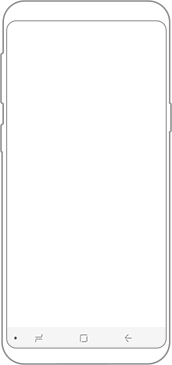This detailed sketch features the outline of a mobile phone set against a predominantly white background. The sketch is rendered in various shades of grey. The exterior edge of the phone showcases subtle ridges that delineate pressable buttons along the side. On the left side of the phone, there are two slightly protruding sections near the upper-left corner, likely indicating volume buttons, with the top section being slightly larger than the bottom one. 

On the right side, there's a similar indentation, possibly representing a lock screen button. Inside the outer outline, there's another grey outline demarcating the phone's screen. At the bottom of this inner outline, a greyed section appears almost rectangular but features rounded bottom corners to match the screen's rounded outline.

This section contains several small icons that resemble functional buttons. On the left, there's a small solid dot. Next to it, two lines are displayed, with the bottom line having a tail that curls downward and the top line having a tail that curls upward. In the center, there's an outlined square, while on the right, an arrow pointing to the left is visible. The interior screen space is entirely white, matching the overall white backdrop and emphasizing the sketch's grey outlines. All in all, this image represents a detailed, grey-scale sketch of a mobile phone's outline and basic button layout.